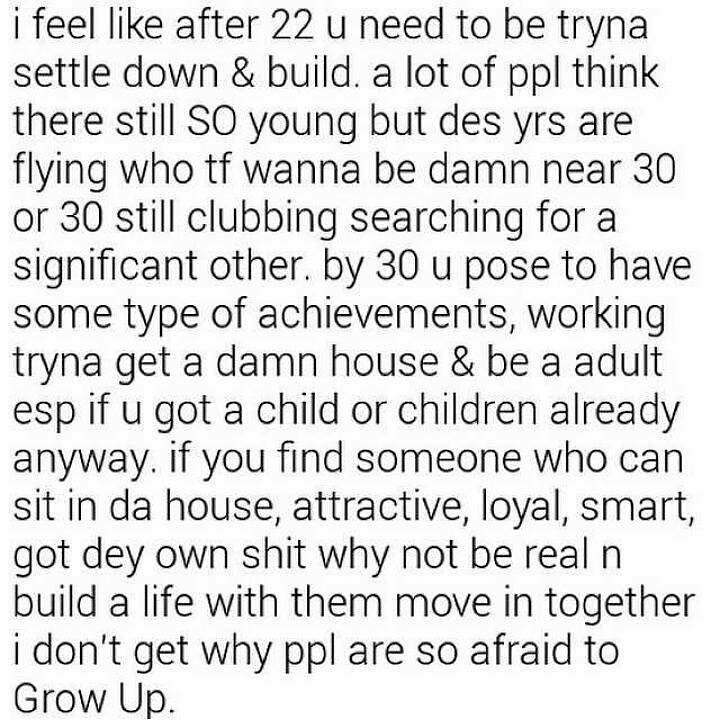The image features a white background with black text styled like a social media post or text message. The text reads: "I feel like after 22 you need to be trying to settle down and build. A lot of people think they're still so young, but those years are flying. Who the fuck wants to be damn near 30 or 30 still clubbing, searching for a significant other? By 30, you're supposed to have some type of achievements, working, trying to get a damn house and be an adult, especially if you already have a child or children. If you find someone who is attractive, loyal, smart, and has their own shit, why not be real and build a life with them? Move in together. I don't get why people are so afraid to grow up." The text is filled with colloquial abbreviations and informal language, reflecting a candid and direct message about maturing and settling down.